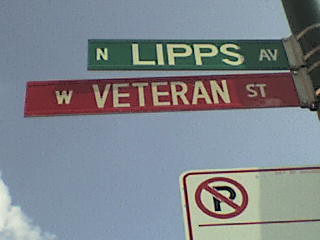The image captures an upward view on a clear, pale blue sky with a few white clouds drifting in the lower left corner. Central to the composition are three street signs affixed to a wooden pole that extends from the lower to the upper right corner. The topmost sign, set against a green background, reads "N Lips Avenue," indicating North Lips Avenue. Below it, a sign with a red background displays "W Veteran Street," denoting West Veteran Street. Additionally, a white "No Parking" sign is situated towards the lower right corner, completing the assembly of street markers at this intersection.